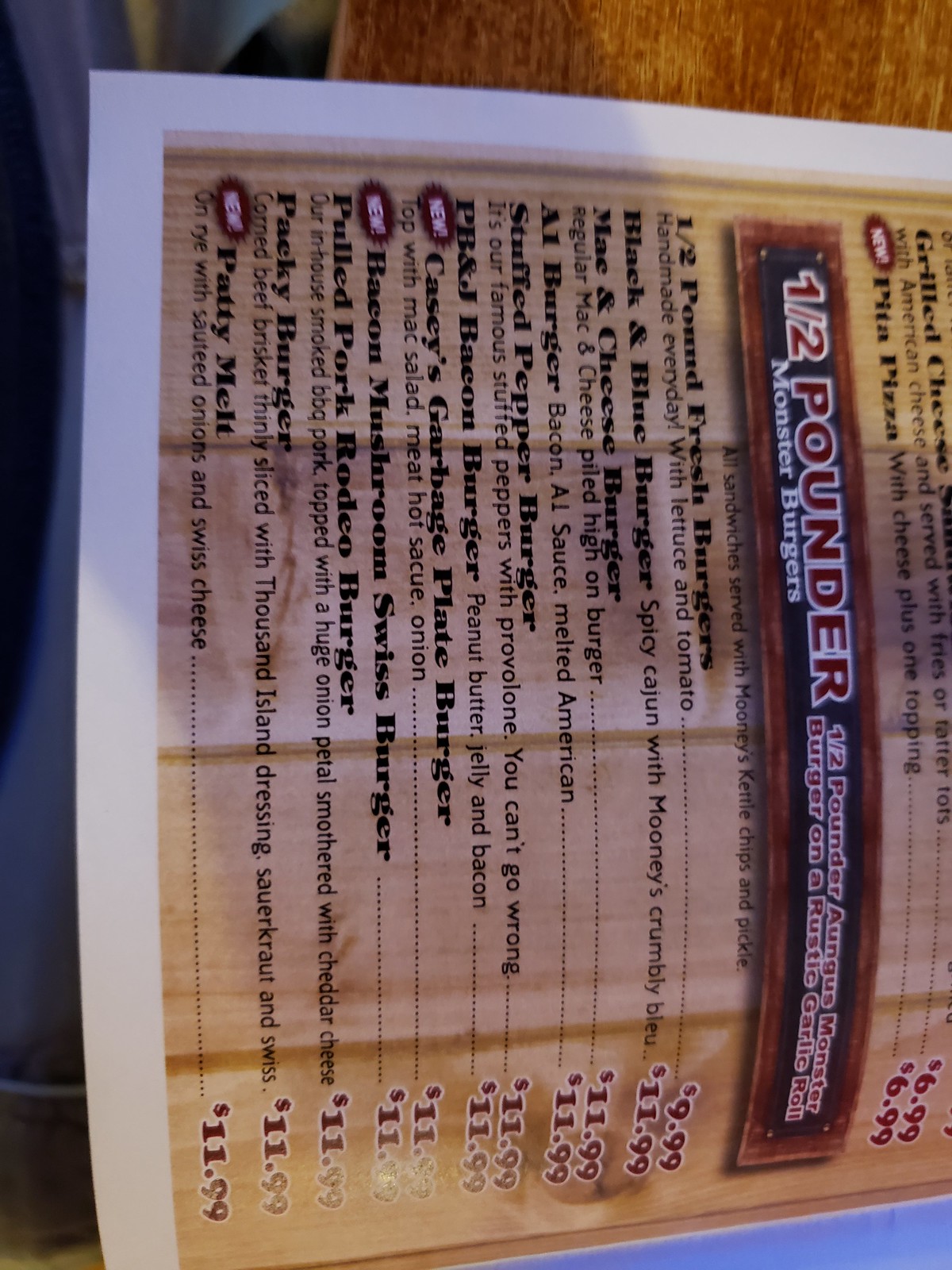The image in question depicts a menu, viewed from the side due to its current portrait orientation. For optimal readability, this portrait image should ideally be rotated 90 degrees counterclockwise.

The menu, which occupies the majority of the frame, features a white border and extends beyond the right edge of the image, making a significant portion of it not visible. The primary focus within the visible section is the "Quarter-pounder" and "Half-pounder" burger sections.

Prominent towards the middle of the image is a banner-like strip with a brown border and a black background. The text within this banner is formatted in vivid red fonts and reads "Half-pounder" followed by "Half-pounder" again in red. Notably, a typo appears here, as it says "Aungus Monster Burger" instead of the intended "Angus Monster Burger," all written in red text on a Rustic Garlic Roll. Beneath this title, "Monster Burgers" is inscribed in smaller white font.

A list of burgers is displayed under this section. Each burger's name is formatted in bold black text, while the descriptions are written in standard black text. For instance, the first item on the list describes a burger as "half a pound fresh burgers, handmade every day with lettuce and tomato," accompanied by a price in an unspecified currency that might not necessarily be USD.

The listed burgers include:
1. Black and Blue Burger
2. Mac and Cheese Burger
3. A1 Burger
4. Stuffed Pepper Burger
5. PB&J Bacon Burger
6. Casey's Garbage Plate Burger
7. Bacon Mushroom Swiss Burger
8. Pulled Pork Rodeo Burger
9. Paki Burger (spelled "P-A-C-K-Y")
10. Patty Melt

Beside this, above the burger section, the menu also lists other items such as "Pita Pizza" and "Grilled Cheese," but these items are barely visible as they extend off the menu's right edge.

Importantly, this menu rests on a brown wooden table, adding to the rustic aesthetic of the overall presentation.